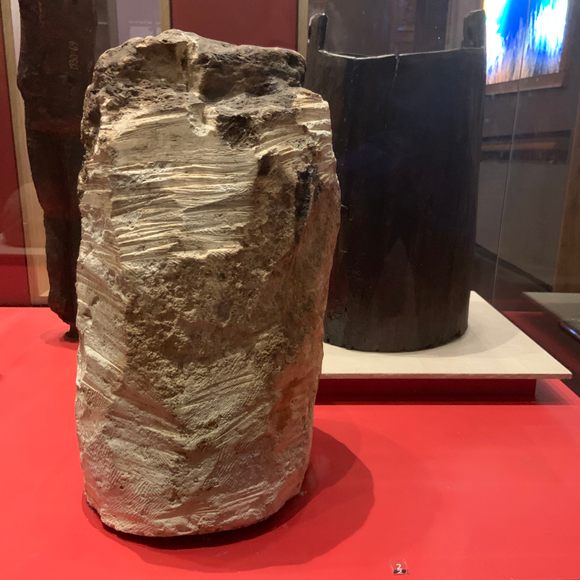The image depicts a cylindrical rock formation, possibly a core sample, on display, reminiscent of a museum setting. The rock, which appears to be partially shaved and transitions from white at the bottom to brown and black at the top, sits on a red display table. Encased in glass, the exhibit reflects light off its surface, obscuring some background details. To the right, there is a metal device, likely used to retrieve or hold the sample, suggesting a scientific context for its exhibition. A black shield, possibly an unrelated exhibit, is placed nearby on a white platform. The floor beneath the rock is distinctly red and the background features indistinct elements, including reflections and fragments of what might be a screen or artwork, indicating a somewhat hurried snapshot of the scene.